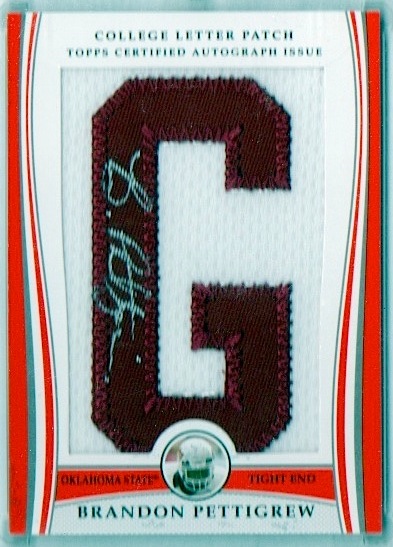This image depicts a detailed trading card, specifically showcasing an autograph card of Oklahoma State Tight End, Brandon Pettigrew. The card has a College Letter Patch prominently featuring a stitched letter "G" at its center, on a white background. The letter is horizontally signed in blue ink by Brandon Pettigrew. The top of the card reads "College Letter Patch" and "TOPS Certified Autograph Issue." Towards the bottom, the card clearly identifies "Oklahoma State Tight End" and "Brandon Pettigrew" in green text. The card's edges are decorated with a light bluish-green border and vertical reddish-orange stripes. The overall design incorporates a mix of white, orange, and light blue colors, along with a small circle featuring an image of a helmet.